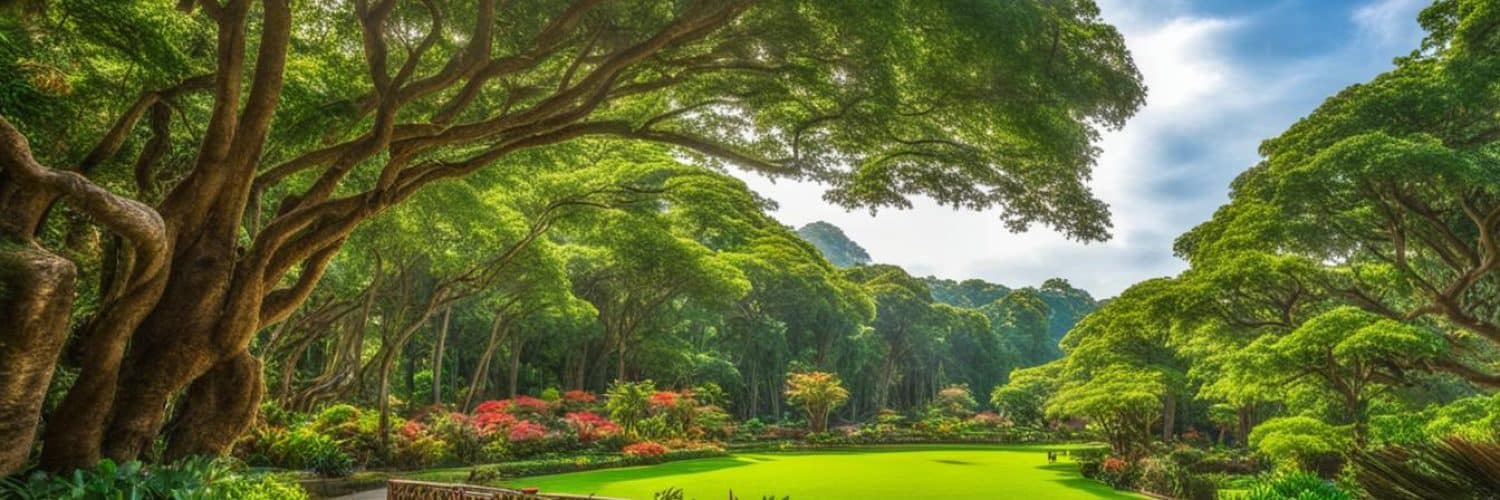This intricate and vibrant painting of a pastoral scene captures a lush, fairy-tale landscape predominated by rich greens. Central to the image is a sprawling field of green grass, flanked by forests of mature, gnarly trees with thick trunks and endless squiggly branches. A particularly striking tree on the left has a mushroom-shaped canopy, with leaves only at its tippy top. Closer to the viewer, a beautifully landscaped garden boasts red and pink flowers amidst verdant foliage. Hidden within the field, a tiny animal—possibly a dog or deer—adds a touch of life and intrigue. The sky, glimpsing through the trees in the background, is a serene blue adorned with white clouds. The entire scene is painted in landscape mode, extending longer than a typical A4 size, evoking a sense of depth and tranquility.